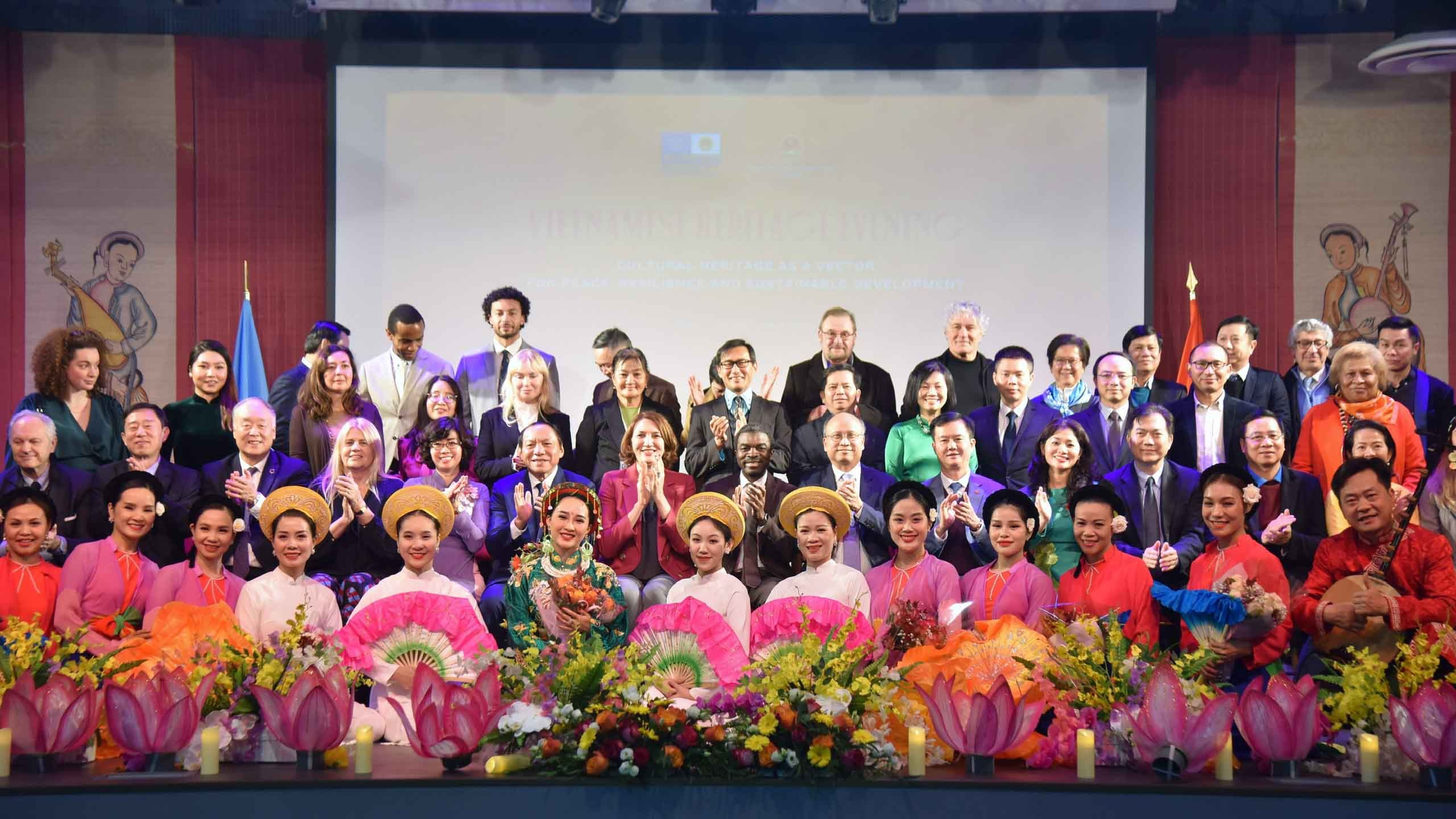This indoor color photograph showcases a well-coordinated group of people posed in four rows. The front row features predominantly women adorned in traditional Asian attire, including vibrant dresses and circular light brown hats, their hair neatly tied into buns. Some women are holding pink fans with green accents, and a striking number of pink flowers and diverse floral bouquets decorate the foreground. A man on the far right of this row holds a guitar-like stringed instrument, adding a musical element to the scene.

Behind them, the second row comprises a mix of men and women in formal wear such as dresses and suits, all appearing to applaud with visible mid-clap hands. The third and fourth rows follow a similar mix, standing and smiling for the camera. Throughout these rows, the attire continues to be formal and celebratory.

Flanking the group on either side are red curtains, with a blue flag on the left and a red flag on the right, creating a regal atmosphere. A projection screen forms the backdrop, faintly displaying what appears to be "Vietnamese Heritage Evening" among other indistinct text. Also present on the back wall are painted images of women in colorful traditional outfits and hats, enhancing the cultural essence of the scene.